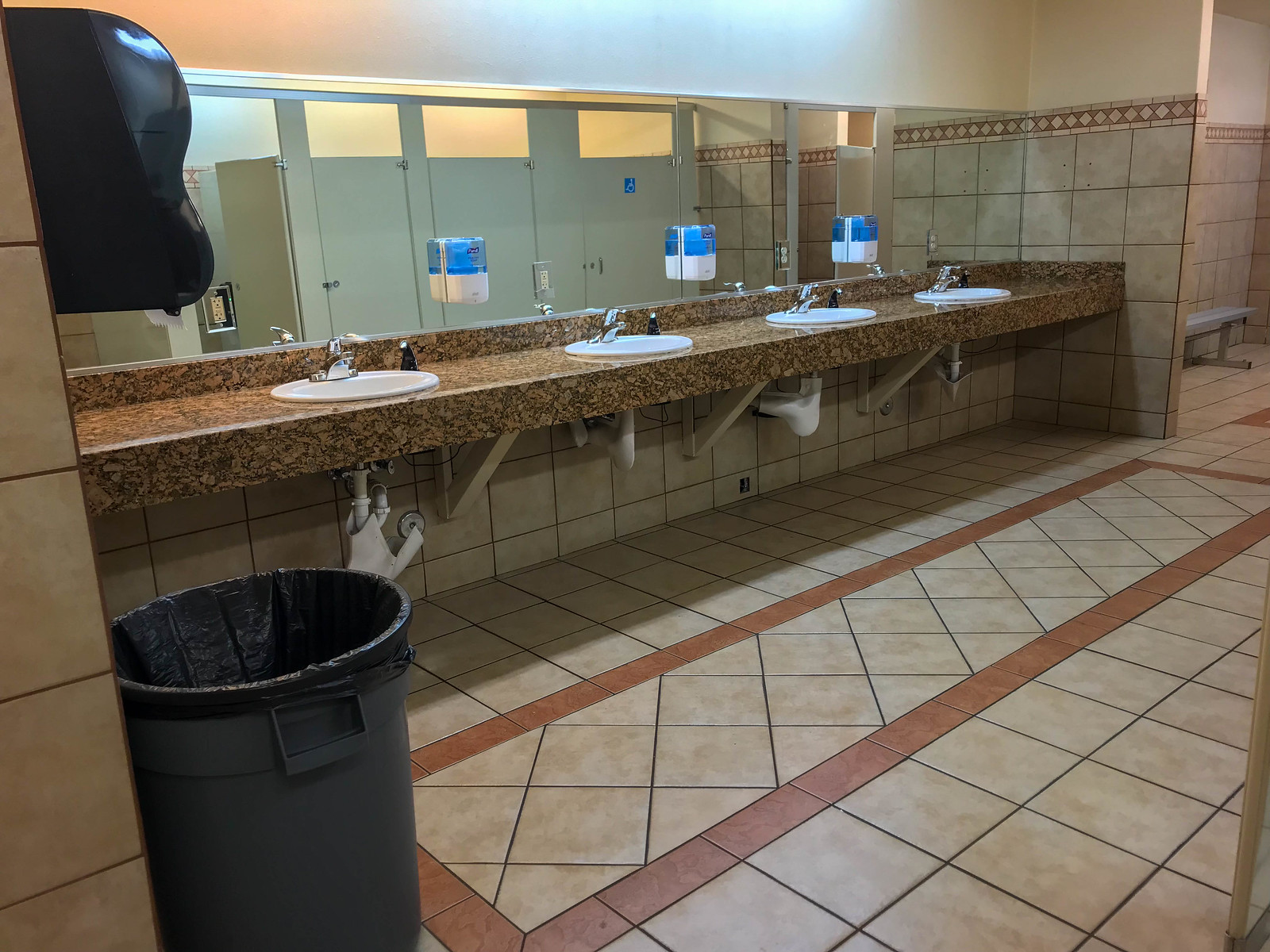This is a color photograph of a public restroom, captured from the entrance. The restroom features a floor made of light brown tiles with dark brown grout, accented by a rectangle of orange tiles. The walls are adorned with light brown tiles that transition to white at the top. Prominently, along the left side of the image, a brown marble-like ledge hosts four round white sinks with stainless steel faucets, and visible plumbing beneath. Above these sinks is a long mirror extending across the countertop, reflecting light tan bathroom stalls—one of which displays a blue handicap access sign. Affixed to the mirror are three soap dispensers with blue tops and white bottoms. In the upper left corner of the image, a black towel dispenser is mounted above a tall black trash can containing a black trash bag. Toward the far right corner of the image, a bench is partially visible. This realistic photograph meticulously captures the functional yet simple design of a public bathroom.